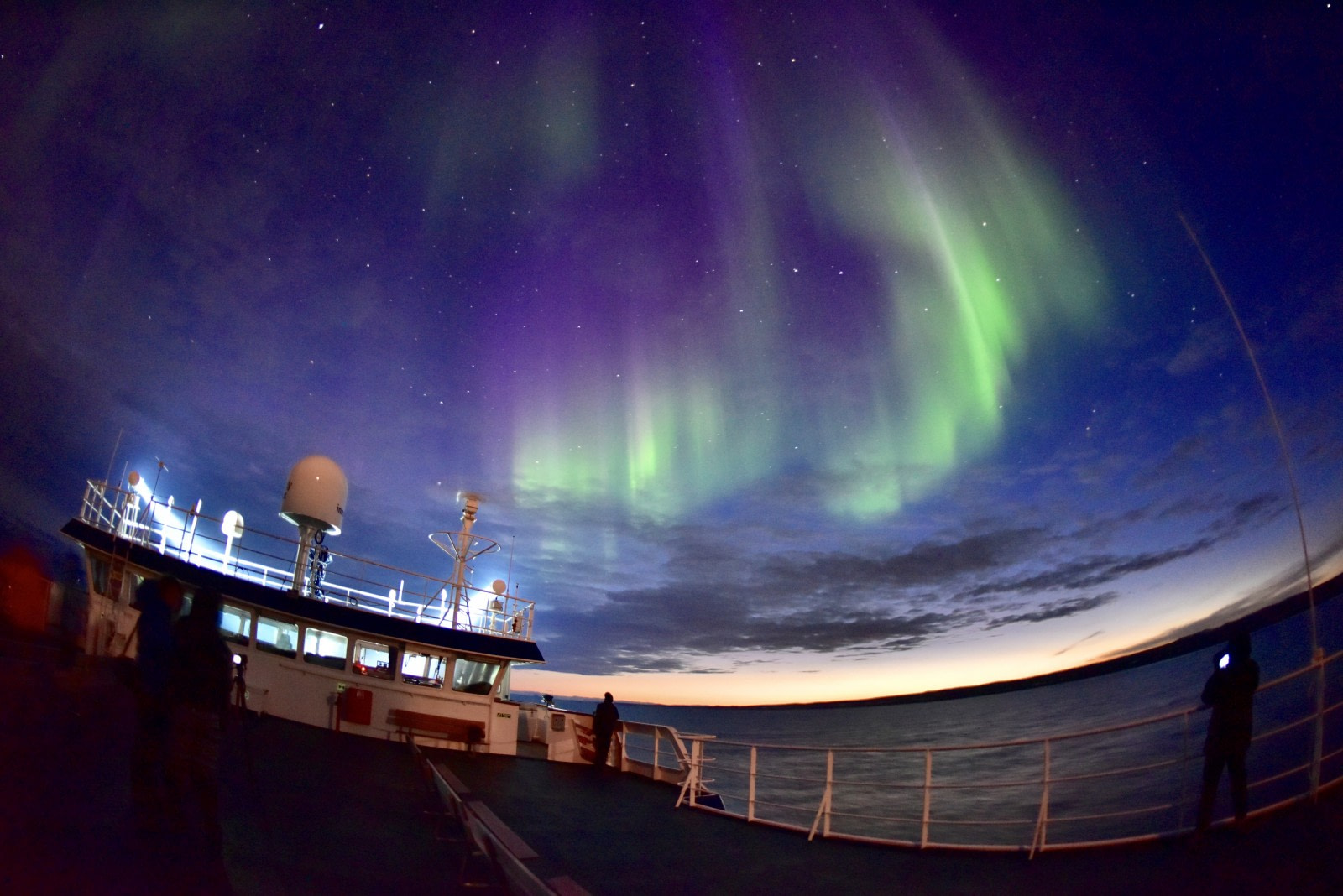The photo captures the mesmerizing Aurora Borealis lighting up the nighttime sky with vibrant green and purple streaks. The sky is a dark canvas of deep purples, blues, and blacks speckled with white stars, and a hint of low sunlight lingers on the horizon, suggesting a high northern latitude. The scene unfolds on a large, white-painted ship, possibly a ferry or cargo vessel, anchored on the calm ocean. The ship's deck features white metal guardrails, a captain's deck with windows, and several satellite dishes. Silhouetted figures, likely passengers or crew members, are visible on the deck, some capturing the natural spectacle with their cameras. The overall atmosphere is one of serene awe, as the celestial dance of the Northern Lights commands attention from all aboard.